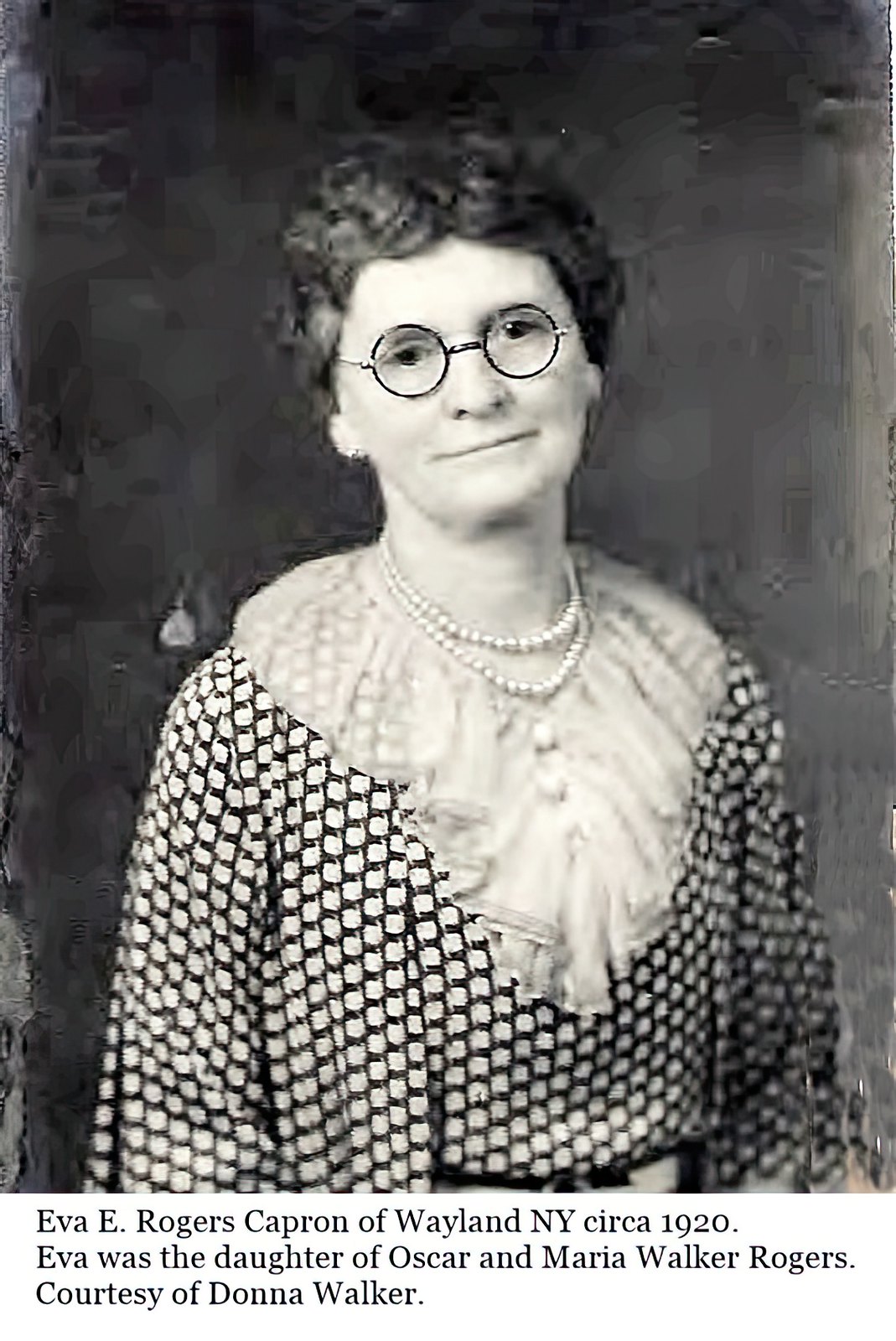This is a black-and-white professional photograph from around 1920, depicting Ava E. Rogers Caprone of Wayland, New York. Ava, a Caucasian woman in her 40s or 50s, stands confidently against a smudged black and gray background. She has short, curly dark hair and wears perfectly round rimmed glasses. Her attire features a distinctive black and white dress with a herringbone pattern, reminiscent of a checkered design, adorned with a delicate lacy collar and two strands of pearls around her neck. The photograph's caption reads: "Ava E. Rogers Caprone of Wayland, New York, circa 1920. Ava was the daughter of Oscar and Maria Walker Rogers, courtesy of Donna Walker."